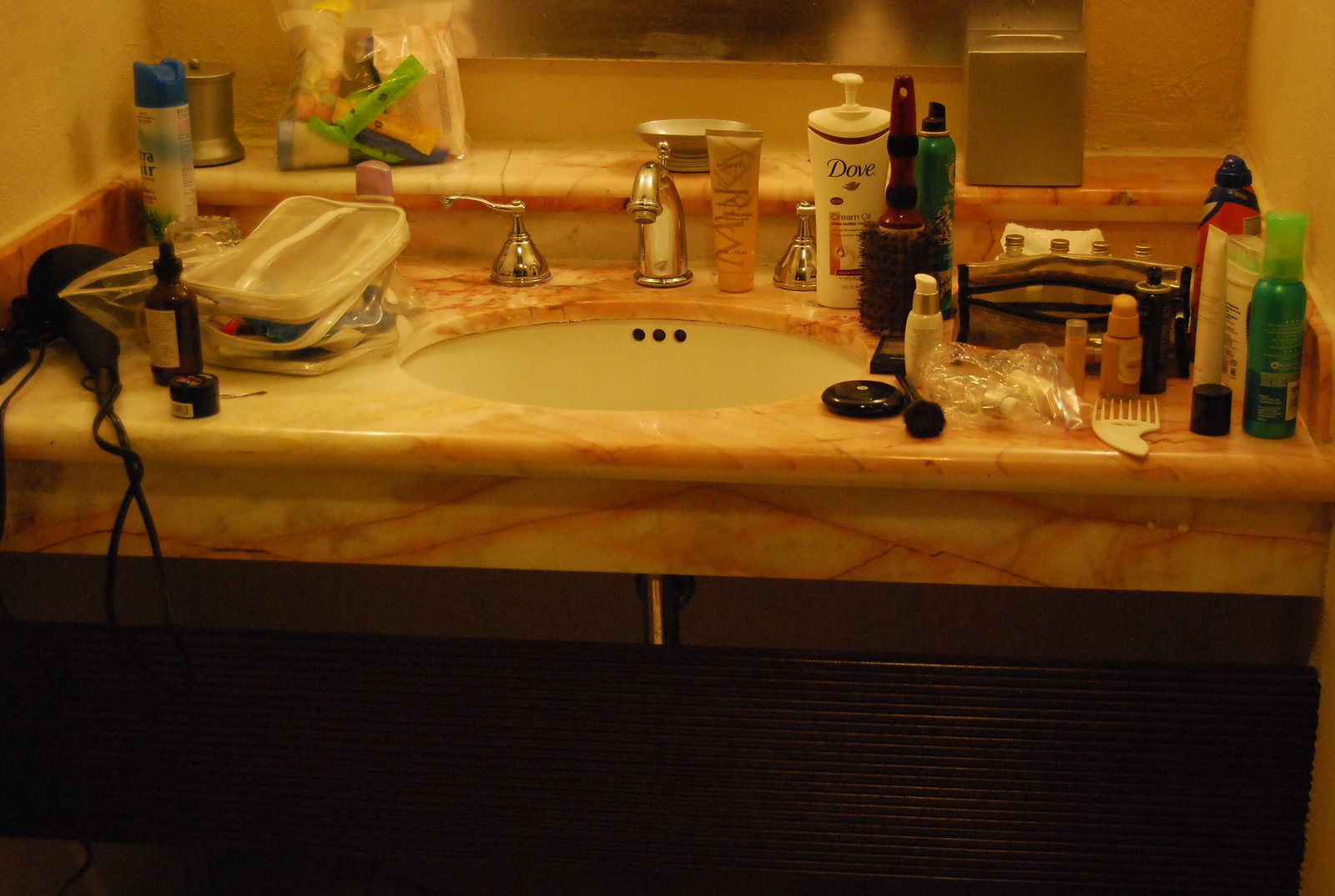The image showcases a bathroom vanity with a round white ceramic sink that includes three drain holes situated directly beneath the spout. The vanity features separate hot and cold water knobs flanking a central spout. The mirror behind the sink extends the view of the cluttered countertop, which is laden with various bathroom products. Near the right-hand cold water handle, a pump bottle of Dove soap is visible. Between this handle and the spout, there's a tube of an unidentified bathroom product. To the left, the countertop displays a range of items including a blow dryer, a cylindrical can of hairspray with a blue top, a hair pick, make-up pads, and assorted containers filled with beauty and hygiene products.